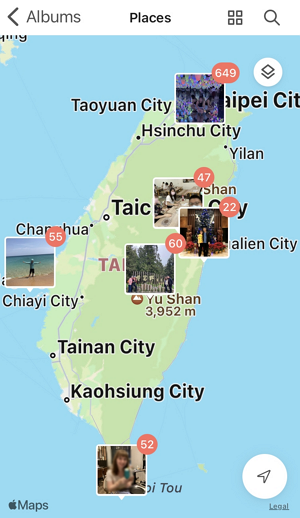The image is a detailed screenshot of a digital map showcasing an island with several labeled cities, including Chai City, Taiyan City, Taipei City, and Yilan City. Within the map, there are specific pinned locations marked with red circles containing numbers such as 22, 47, 52, and 55. Each marked location is associated with profile pictures of different individuals, suggesting the presence of users or friends mapped to these areas. In addition, the map features an icon of a circle with a black arrow inside, likely representing a navigation or location pointer. The detailed city labels and user profiles create an intricate network of connections within this virtual island map.